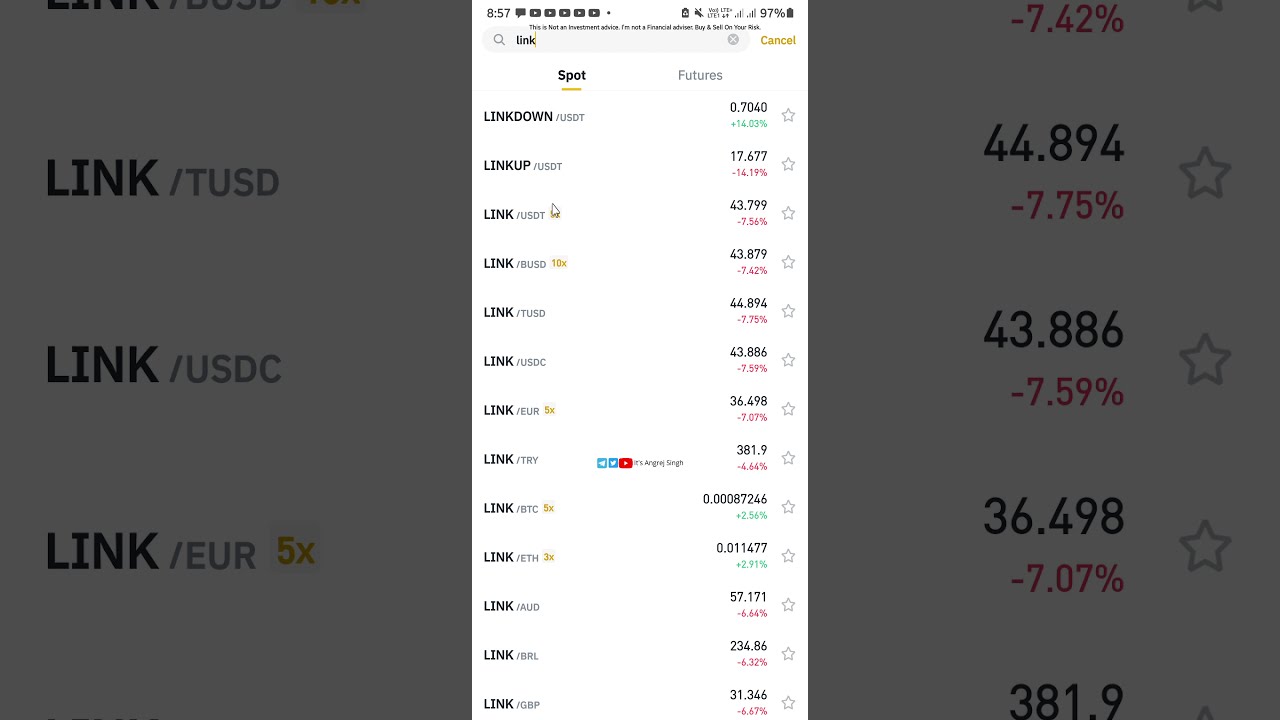The image displays a cell phone screen capture of a financial app, centered within a vertical white rectangle against a dark gray shaded background. The time on the phone is 8:57, with the battery at 97%. At the top of the screen, the search bar contains the word "Link." Below the search bar, there are two tabs labeled "Spot" and "Futures," with "Spot" highlighted in bold black text. The app features a detailed table of financial assets, with left-aligned names of various currencies and cryptocurrencies including the U.S. Dollar, Euro, Bitcoin, Ethereum, and others, paired with their corresponding prices and percentage changes on the right. Notably, the data sections list "Link/TUSD," "Link/USDC," and "EUR 5X" on the left, and respective prices alongside percentages such as "44.894, -7.75%", and "43.886, -7.59%" on the right, each followed by a star symbol. The dark filter overlaying the zoomed-in and zoomed-out forms of the screen provides a focused yet stylistically subdued view of currency rates within the app. It remains unclear whether this screen reflects a user's personal portfolio or merely a reference table being consulted.